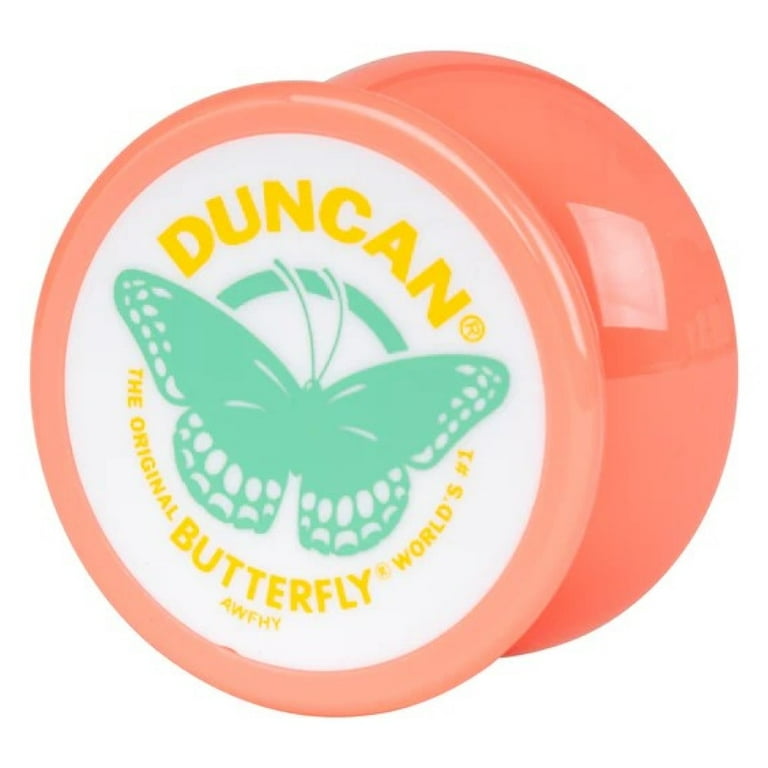This detailed close-up photograph showcases a nostalgic yo-yo, prominently featuring the brand "Duncan" in bold yellow letters with an ® trademark symbol beside it. Centered on the circular label is an illustration of a green butterfly, which bears white spots near the edges of its wings and is encircled partially by a green arc above. The text beneath the butterfly reads "the original butterfly, world's number one," also in yellow font. This yo-yo, reminiscent of childhood memories, is strikingly pink with a shiny, bulbous surface that reflects light, highlighting its vibrant color. Although the string is not visible, the image captures the yo-yo's charm and the sentimental value it holds for those who cherished it in their youth.